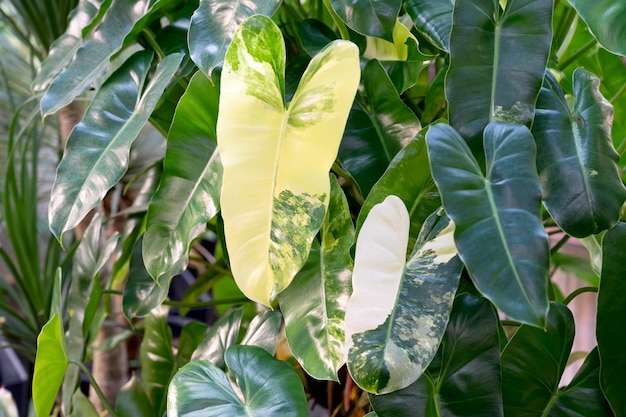The photograph captures a vibrant outdoor scene bathed in sunlight, showcasing a variety of large, heart-shaped leaves with striking color variations. Dominating the center is a prominent leaf with a creamy white and green variegation, displaying an elongated heart shape and a distinct central vein. To its immediate right is another variegated leaf, predominantly white on the upper part with green tinges. Surrounding these central leaves, a mix of bright and dark green foliage extends outward, their glossy texture hinting at the influence of the sunlight that illuminates the left side of the image. The leaves on the right appear darker and more plastic-like due to being in relative shade. An off-white wall partially frames the right side of the image, while the left side is accented by grassy-shaped plants, adding to the tropical ambiance. The entire scene conveys a lush, sunlit environment with a subtle play of light and shadow.